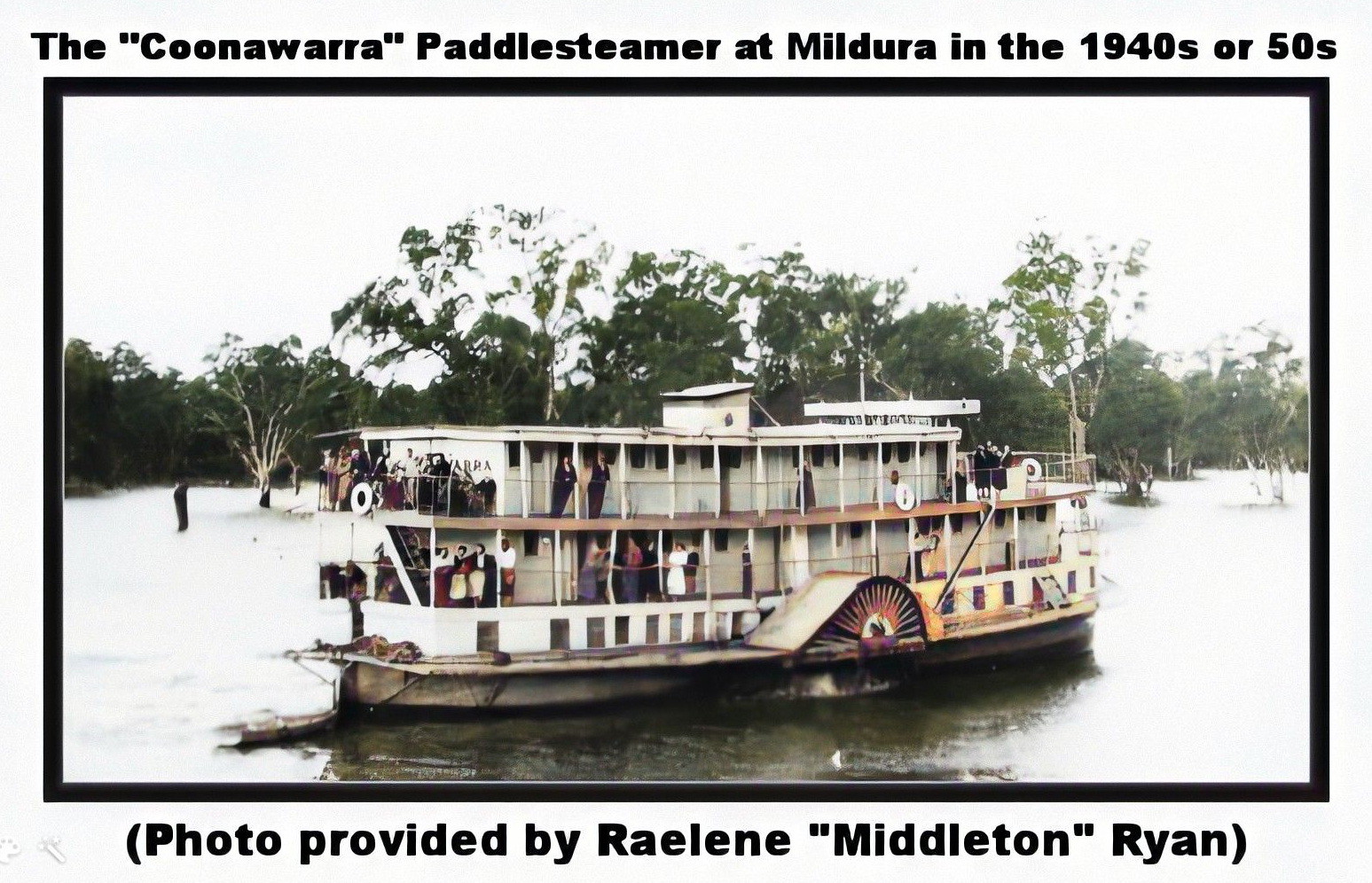This historical photograph, framed in a white outer border with a black inner border, depicts the "Kunawara" paddle steamer at Mildura during the 1940s or 50s. The caption at the top is printed in bold black, and it reads, "The Kunawara paddle steamer at Mildura in the 1940s or 50s." Below the image, another bold black caption states, "Photo provided by Raylene Middleton Ryan." The paddle steamer, which appears to have been color-edited, features two levels with visible railings. Passengers are seen on both decks, some looking out at the water while others wave. The boat is predominantly white, with a large paddle wheel located centrally along its hull and a life preserver attached to the upper deck railing. Prominently displayed on the side is a swan logo. The steamer is navigating through a murky green river surrounded by densely packed, leafy trees and a bright, reflective sky that indicates daylight.